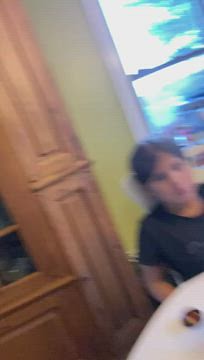The image depicts a blurred, vertically-oriented photo taken inside a house, likely on an older phone, featuring a young person sitting at a round, white table. The individual, who appears to be a child or teenager with short to medium-length brown hair, is wearing a dark, short-sleeved shirt and is seated in front of a window with a white frame. Sunlight streams through the window, illuminating blurred trees and a hint of blue sky outside. The wall behind the child is yellow, and to the right, there is a tall wooden armoire or cupboard, possibly with glass doors that may contain dishes. The child's arms are visible, resting on the table, but their hands are obscured. A small, indiscernible object sits on the table, adding to the overall sense of mystery in this nostalgic, low-quality photograph.